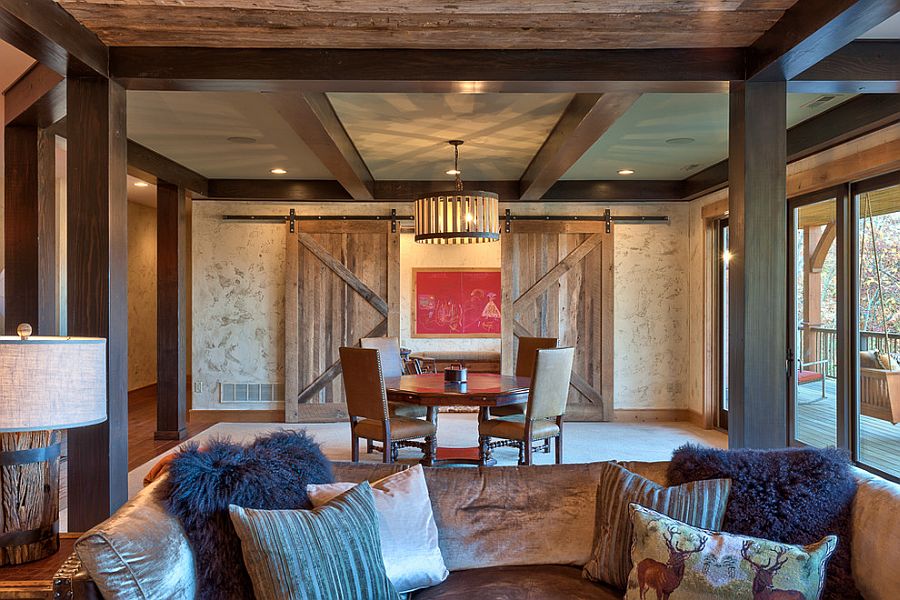This indoor photograph captures a cozy and rustic living space that appears to combine the living room and dining area. Dominating the foreground is a brown leather couch adorned with six throw pillows: two fuzzy blue pillows, two brown and white striped pillows, a single white pillow on the left, and a larger pillow featuring a print of deer with prominent brown antlers on the right. To the left of the couch stands a wooden table with a lamp shaped like a wooden barrel, topped with a beige lampshade.

In the background, a dining table surrounded by four chairs is visible. The area is illuminated by a chandelier casting a warm and inviting glow. Behind the table, there are large sliding wooden doors, resembling barn doors, that likely lead to another room or pantry. To the left, a hallway is partially visible, while to the right, sliding glass doors open to an outdoor wooden deck. The deck features a wooden swing and a chair, framed by a wooden railing and fences, with trees in the distance adding to the homely atmosphere.